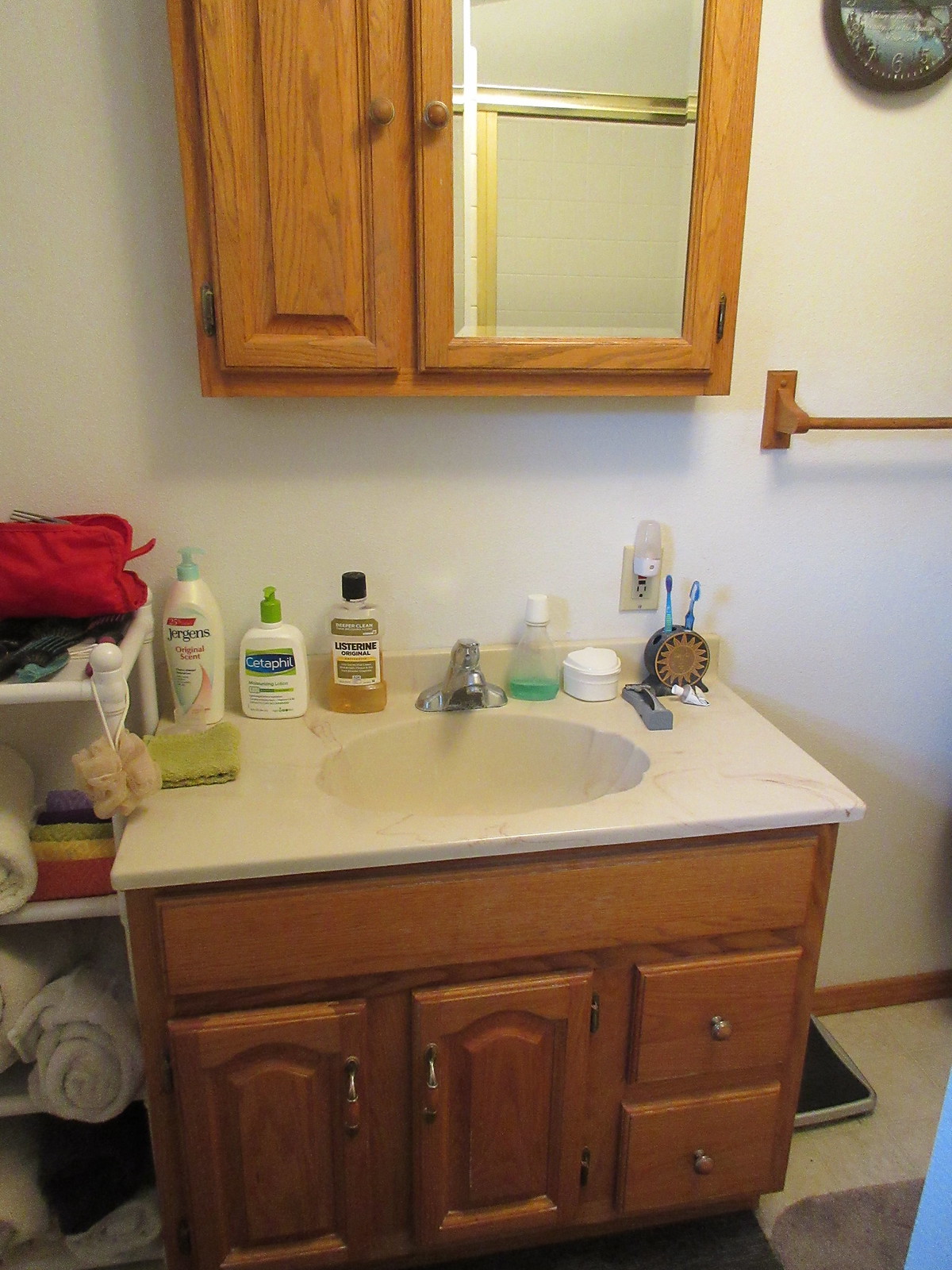The image depicts a slightly dated bathroom vanity, likely from the 1970s or 1980s, constructed from medium light oak wood. The vanity features two drawers on the right side, fitted with what appear to be gold-toned handles, though the exact finish is somewhat indistinct. To the left of the drawers are two cabinet doors, matching the style and hardware.

The countertop is made from a material typical of the era, resembling a solid plastic composite rather than stone or laminate. The circular sink embedded in the countertop is surrounded by a variety of personal care items: Juergens lotion, a bottle of Cetaphil lotion, and a Listerine bottle fill some of the space. To the left, a greenish washcloth is neatly folded, and a silver-toned faucet gleams near a pump bottle containing green liquid. Additionally, a white container with a lid and a nightlight near an electrical socket are visible. A round toothbrush holder contains two blue toothbrushes and a gray-cased razor.

Above the vanity, there is a matching wooden wall unit with two sections. The right section features a mirrored door, while the left section has a plain wooden door. A matching wooden towel rack hangs on the adjacent wall, contributing to the cohesive vintage look. Attached to the left side of the vanity is a white pipe rack, which holds an assortment of washcloths and rolled-up towels, with a scrubbing tool hanging from one corner.